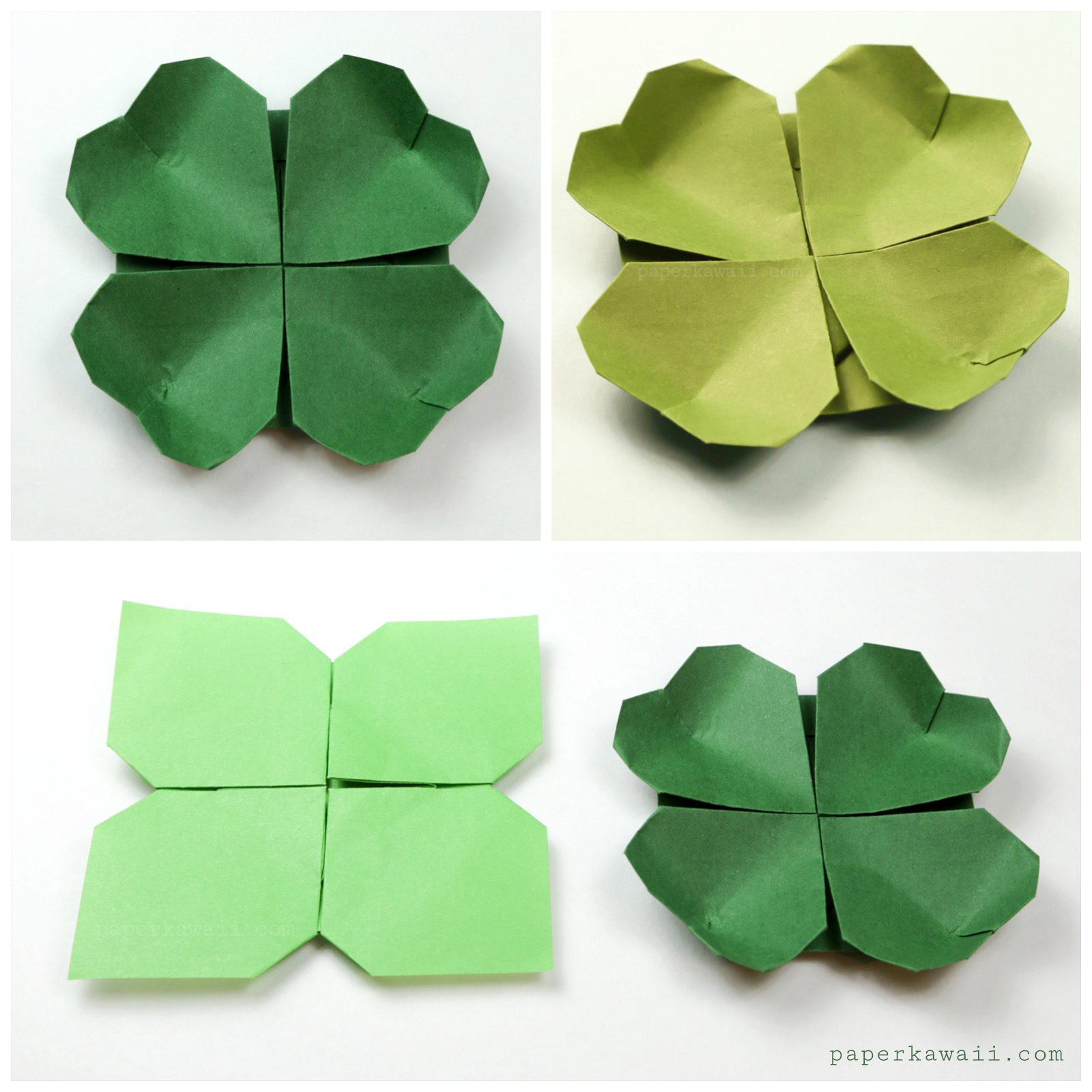This image shows a 2x2 grid of photographs featuring paper clovers, crafted through origami. The top left and bottom right quadrants display dark green four-leaf clovers, each with heart-shaped leaves, accentuating a classic clover design. The top right quadrant features a similar design in an olive green hue. The clover in the bottom left quadrant stands out with its mint green color and stylized X-shaped leaves, differing from the heart shapes of the others. The entire layout has a white background with shadows cast underneath each clover, adding depth. In the bottom right corner, the text "PAPERKAWAII.COM" is printed in black lettering.